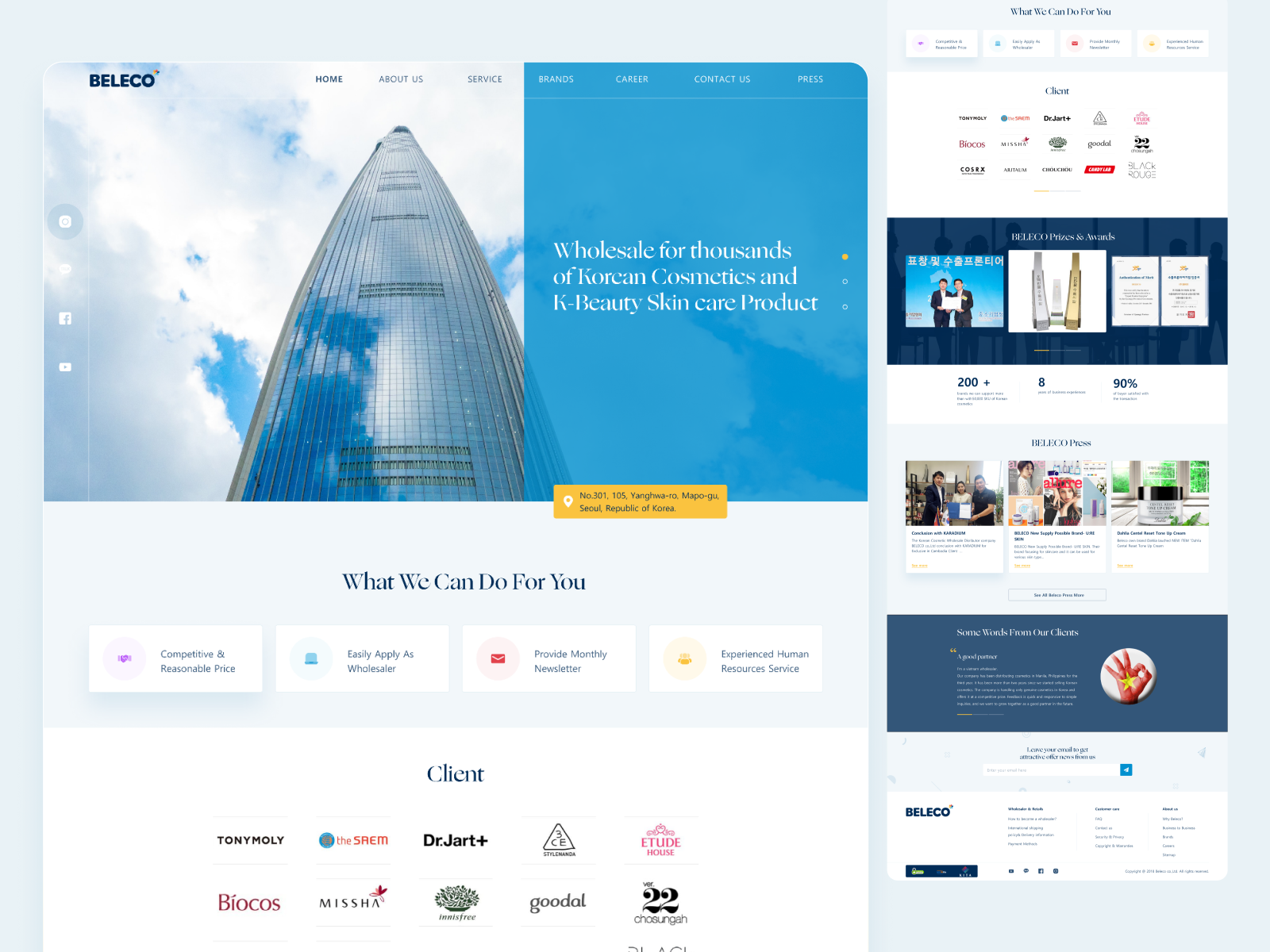The homepage of Belleco, an online platform for wholesale Korean cosmetics and K-beauty skincare products, features a striking main image of a tall, modern building with sleek, reflective windows that create a mirror-like effect. The photograph captures an upward perspective from the ground, emphasizing the building's immense height as it reaches towards the sky, with clouds visible above.

To the right of the main image, a bold blue banner highlights Belleco’s offerings: "Wholesale for thousands of Korean cosmetics and K-beauty skincare products." Beneath this banner, key benefits are listed, including competitive and reasonable pricing and an easy application process for wholesalers.

The page also displays a list of notable clients, such as Misha, Bayakos, and Etude, though these names may not be widely recognized. To the right, a small social media feed presents articles and updates from Belleco, although the text is quite small and difficult to read. The overall background of the homepage features a clean, light gray or possibly white color, providing a neutral backdrop that emphasizes the content.